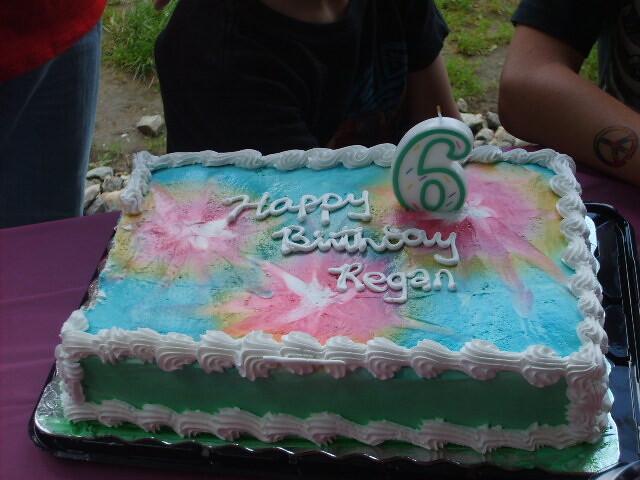The image showcases a detailed close-up of a child's birthday cake decorated with vibrant, tie-dye hues of blue, pink, and yellow frosting, accented with a white border. "Happy Birthday Regan" is elegantly written in white cursive lettering. A prominent number six candle, characterized by a white background and outlined in green, stands tall on top of the cake with an unlit wick. The cake sits on a table draped with a purple tablecloth. Surrounding the cake are three people: two figures wearing black t-shirts—one visible through an arm with a tattoo—and another person in a red shirt and blue jeans. The background reveals a natural setting with a dirt path, scattered rocks, and green leaves, adding to the outdoor birthday celebration ambiance.